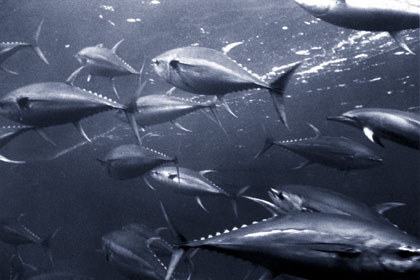This small, horizontal underwater photo, likely taken at an aquarium through glass, captures a dynamic school of silvery tuna swimming in various directions. Illuminated by shafts of light penetrating the water, their sleek bodies and upper fins appear almost white where the light strikes them. The tuna, with their eye-shaped bodies, glisten in a metallic silver hue against the dark, bluish-gray water. The image conveys a sense of bustling underwater life, with countless fish creating an intricate, mesmerizing tapestry within the aquatic environment.